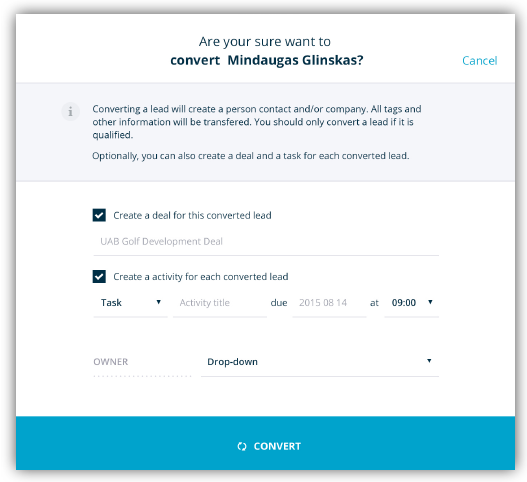The image depicts a rectangular dialog box with a white background, framed by a gray shadowy border that becomes lighter towards the edges. 

At the top of the box, there's a prompt that reads, "Are you sure you want to convert mine doggers Glen scuffs?" Below the prompt, a blue hyperlink labeled "Cancel" is displayed.

The dialog box is segmented into different sections. The next section has a gray background featuring a gray circle with a lowercase 'i' icon to the left. To its right, a message explains the implications of converting a lead: "Converting a lead will create a person contact and/or company. All tags and other information will be transferred. You should only convert a lead if it is qualified. Optionally, you can also create a deal and a task for each converted lead."

Further down, there's another white background section with two checkboxes. The first checkbox, in the middle, is labeled "Create a deal for this converted lead." Below it, an input line reads "UAB Golf Development Deal."

The second checkbox, also checked, is labeled "Create an activity for each converted lead," followed by a text input field labeled "Tasks activity title clue."